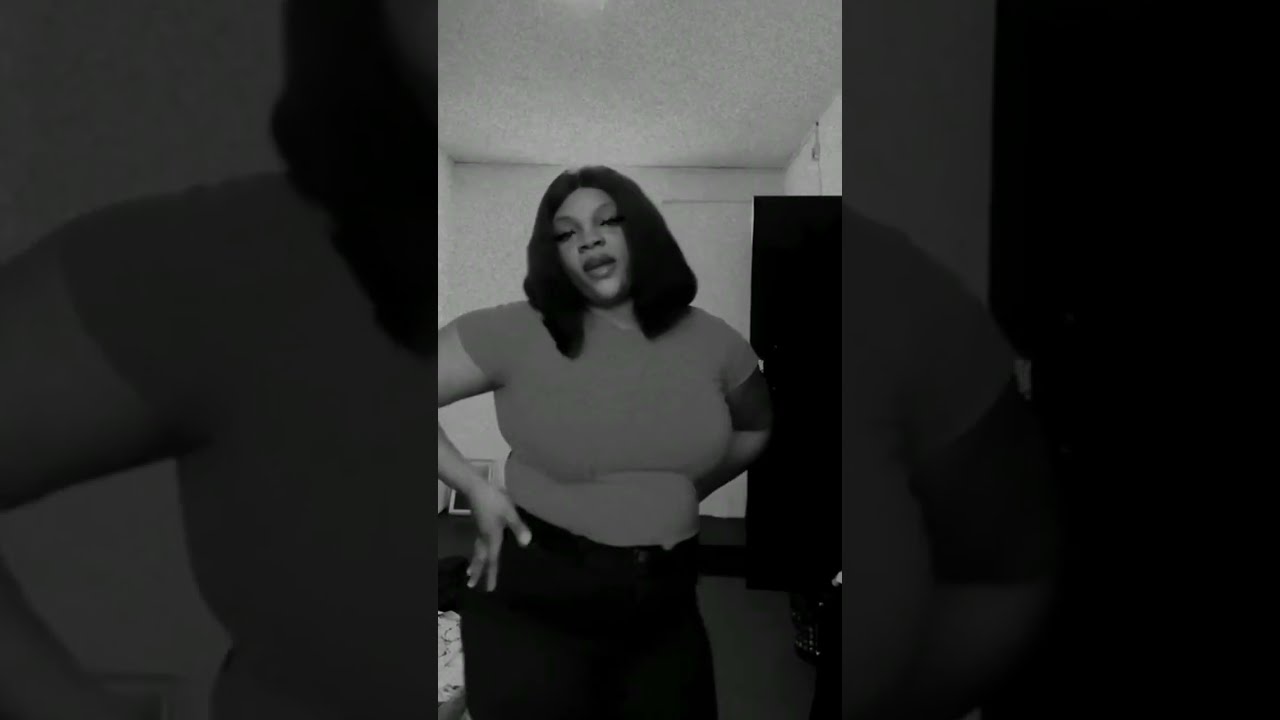This black and white photograph showcases an African-American woman posing confidently with her hands on her hips. She stands centrally in the image, which features a vertical strip of the woman overlain on a background comprised of a darker, close-up repetition of her form on the left and right thirds. She is dressed in a light short-sleeve shirt tucked into black pants, accentuating her curvy figure. The woman has shoulder-length, straight black hair and wears makeup, including fake eyelashes and lipstick, enhancing her striking features. Her expression is both seductive and sassy, suggesting she might be singing, dancing, or perhaps recording an instructional video in what seems to be a room with gray-toned walls. In the background, there’s a dark object that could be a TV and a framed picture with a white border and dark center, adding subtle layers to the scene's domestic setting. The overall composition makes her the focal point, emphasizing her presence and attitude.